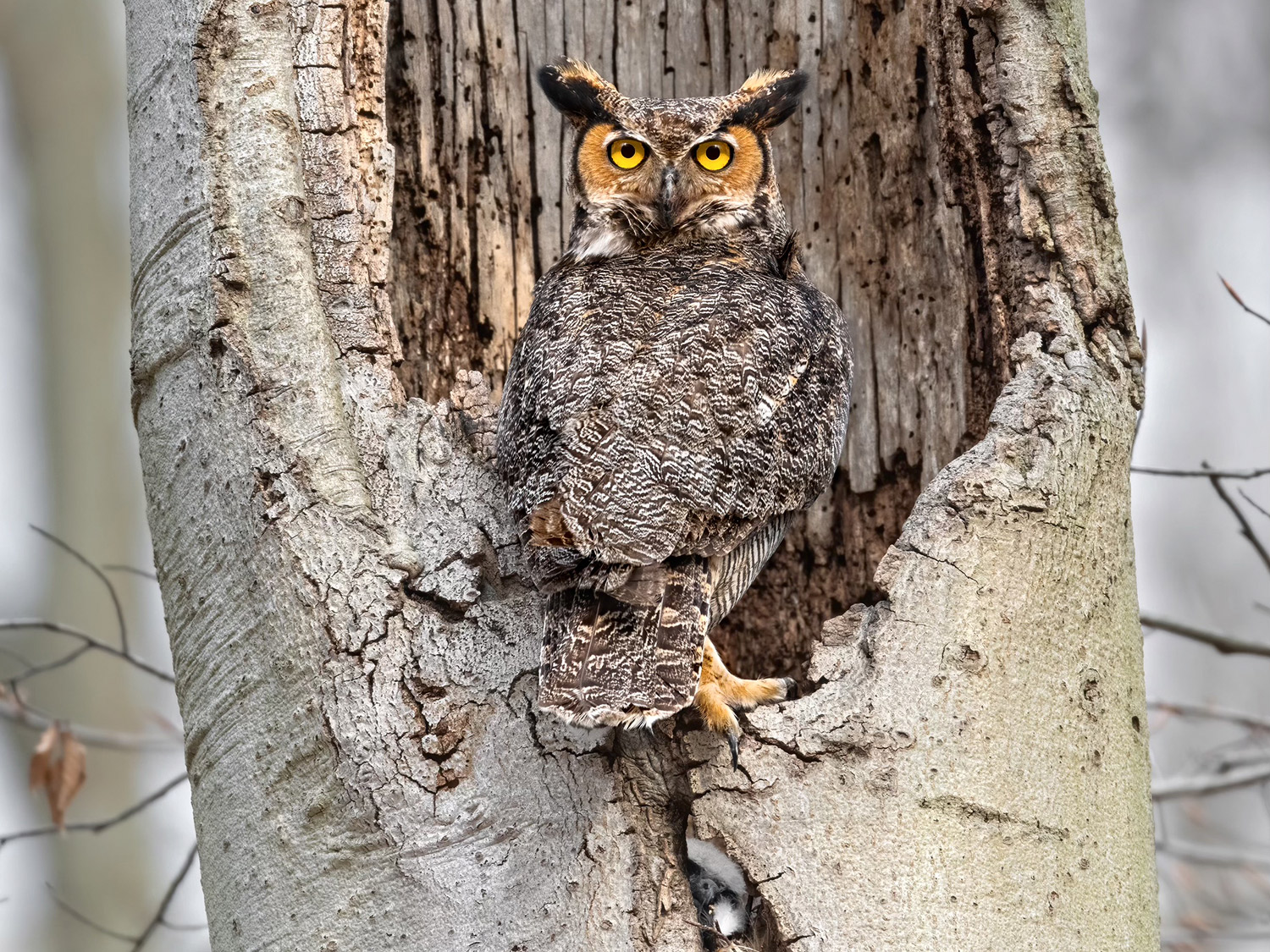This high-quality photograph captures a captivating scene of a brown and gray owl perched in a hollowed-out section of a large, weathered tree. The owl, expertly camouflaged with the tree's bark, is strikingly detailed, showcasing its textured feathers and prominent ear tufts. With its head turned almost 180 degrees, the owl's piercing bright yellow eyes gaze directly at the camera, creating an intense, soul-piercing connection with the viewer. The background is blurred, suggesting a wintry or late autumn day, with exposed branches devoid of leaves and a single brown leaf clinging to a branch in the bottom left corner. The overall image exudes a sense of stark, natural beauty and the quiet resilience of wildlife.